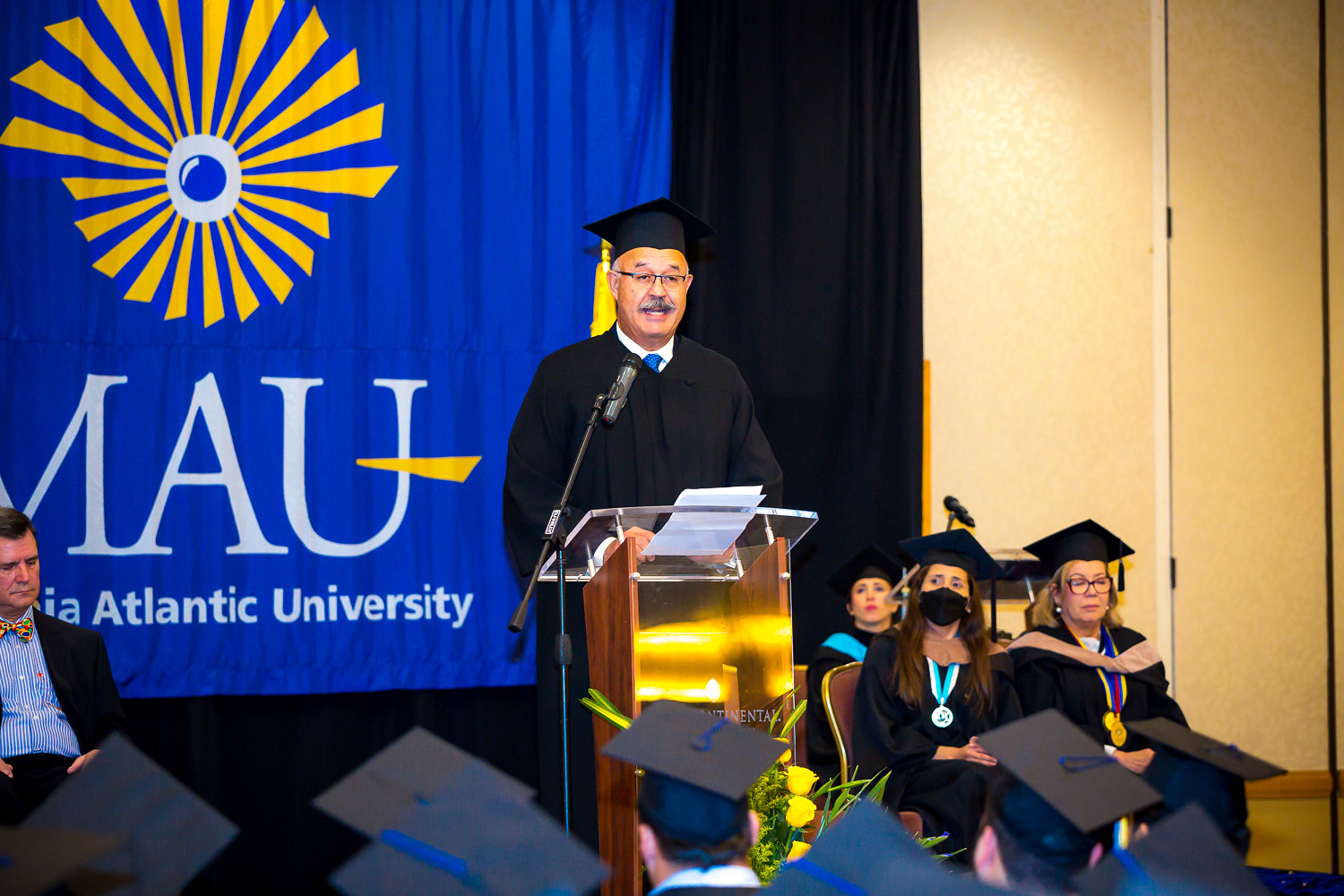In the image, an older man with balding hair, dark eyebrows, a mustache, and glasses, stands at a podium. He is donning a white shirt, blue tie, and a graduation gown, complete with a graduation cap. He appears to be giving a speech at a college graduation ceremony. In front of him, the tops of graduation caps are visible, indicating the audience is made up of graduates with their backs to the viewer.

To the left of the speaker, a Caucasian man in a bow tie, striped shirt, and dark blazer with short hair looks downwards, seated on the stage. To the right of the speaker, three women wearing graduation caps and medallions are seated. 

The backdrop features a prominent black banner adorned with a blue and yellow icon that resembles a sun with rays. In front of this banner, the text in white letters reads "MAU" with "Atlantic University" positioned below it. The setting clearly suggests an indoor college or university graduation ceremony, marked by the formality and the academic regalia of the participants.